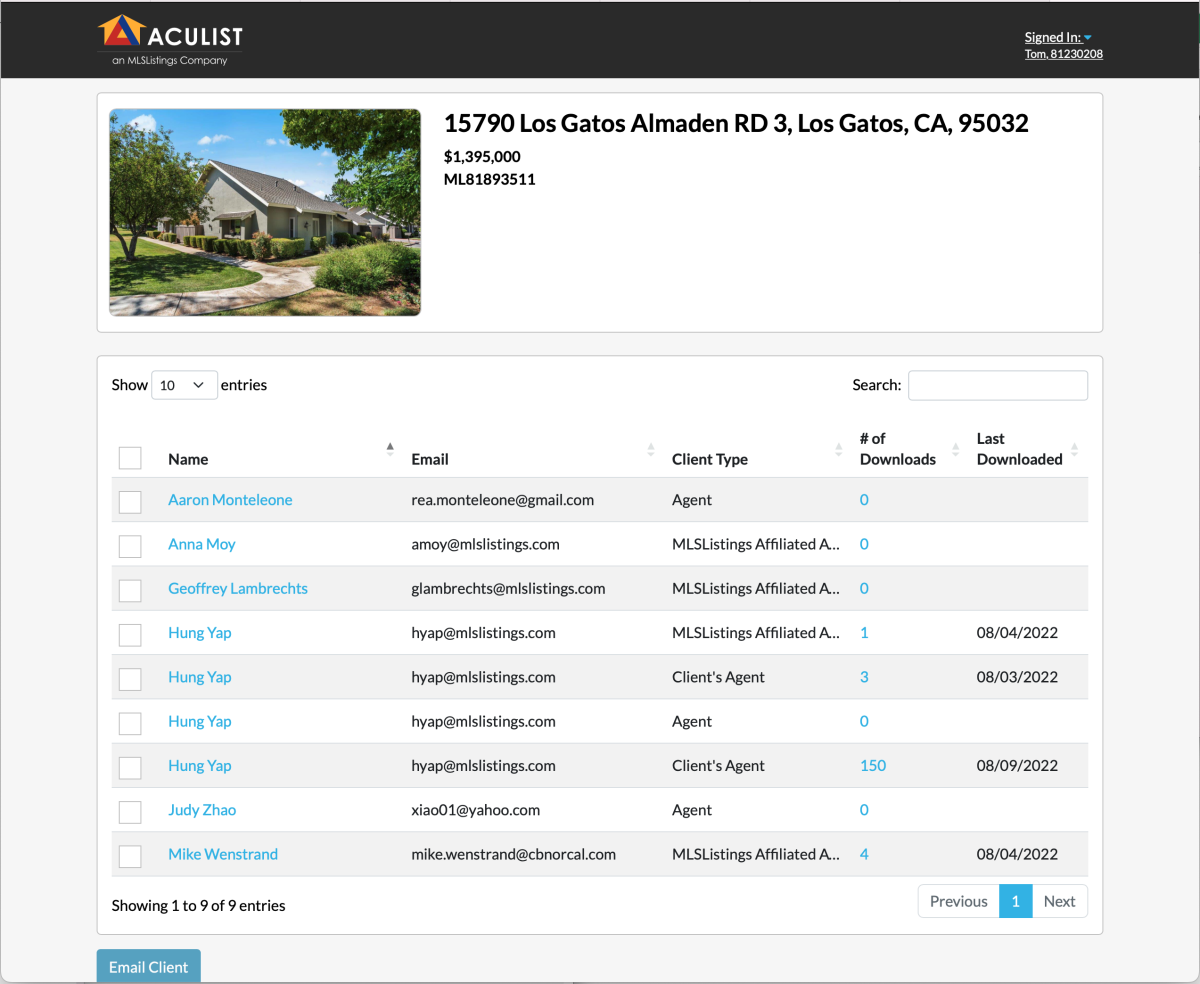Caption: 

"This real estate listing showcases a stunning property located at 1572 Los Gatos, featuring a well-maintained building set against a backdrop of clear blue skies and lush green lawns. The listing, identifiable by MLS number 189593511, is priced at $1,395,000. The property highlights an extensive 2010 entry log, with checkboxes marking off nine entries displayed in a blue rectangular section. Additional details include contact information with the name Tom and the number 81230208, and a reference to the RD3 Los Gatos area with the identifier 1248953032."